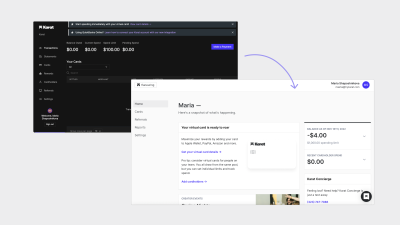The image features two overlapping pages set against a black background. The page on the left, slightly recessed behind the other, has white text and a blue button, partly obscured by the overlapping page. A blue arrow on the left page points to the right page. The right page, white in color, covers the bottom right-hand corner of the left page, with a blue button in the top right corner. Both pages contain text that is too small to decipher. Additionally, the white page displays some numbers, though their context remains unclear. There appears to be a search bar at the top of the black page, though it's indistinct. The backdrop of the image is predominantly white. A black circle with a white box inside it can be seen in the bottom right corner of the white page.